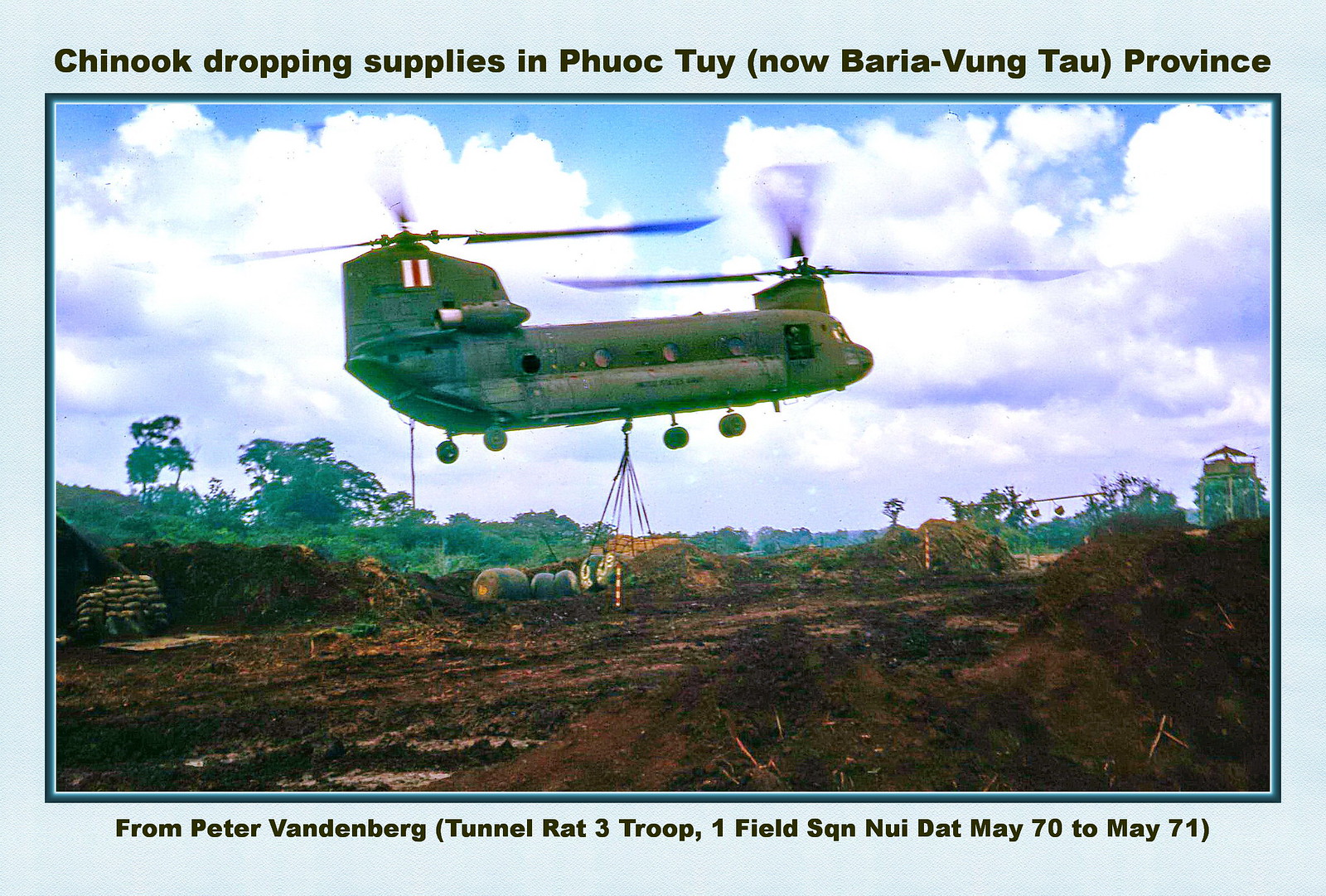This vintage photograph, set against a light blue background with a wide blue border, features a military Chinook helicopter conducting a supply drop during a Vietnam War operation. The helicopter, likely grey or green, hovers low over a muddy, cleared field with disturbed soil in the foreground. The background reveals a jungle setting that has been partially cleared, suggesting possible road construction or a landing zone. Suspended from the helicopter by net-like straps is a package or cargo being delivered to the ground below. A soldier is visible inside the helicopter. The sky is predominantly blue with scattered white clouds, indicating it is a daytime scene, although the day appears cloudy. The text at the top of the photograph reads, “Chinook dropping supplies in Phuoc Tuy, now Baria Vung Tau province,” and the bottom text states, “From Peter Vandenberg, Tunnel Rat 3 Troop 1 Field Squadron, May 70 to May 71.”